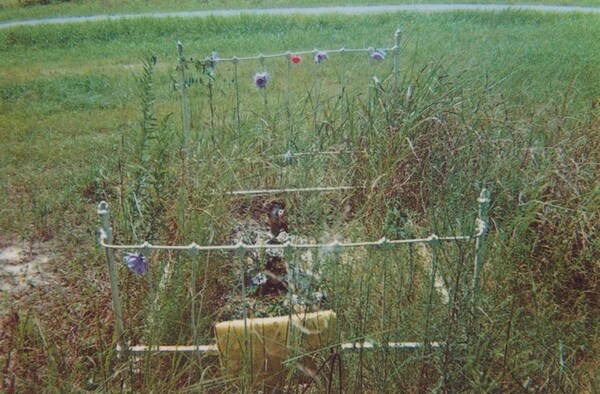In the image, a rusted, white metal bed frame, abandoned and stripped of its mattress, prominently stands in the middle of a grassy field. The bed frame, stained from prolonged exposure to the elements, is adorned with artificial flowers that are wired to the headboard and footboard, creating a whimsical yet forlorn scene. Enveloping the frame are tall, thick weeds about three feet high, with shorter mowed grass seen behind them. The bed frame appears to be reclaimed by nature, as it's nestled in a patch of earth with overgrown weeds crawling up its sides. Beyond the field of tall grass, a narrow gravel road stretches across the background. In front of the bed frame lies a yellow pad with two handles, adding a curious element to the outdoor setup. The entire scene gives a sense of a forgotten place, with the frame humorously resembling a “flower bed.”